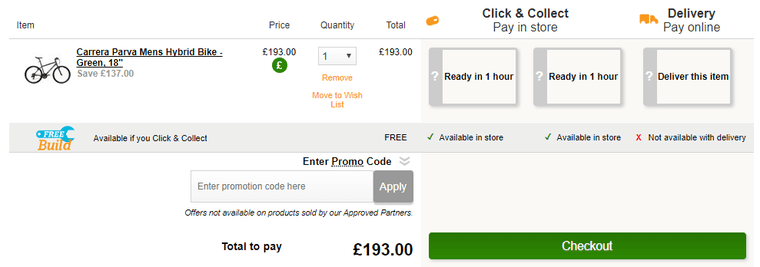The image is a webpage screenshot featuring a listing for a bike. At the top of the page, there's a header labeled "Item". Below this header, there is a digitally rendered image of a bike, specifically, a Carrera Parva men's hybrid bike in green. The description notes that it has an 18-inch frame and mentions a discount, indicating you save £137. The discounted price is prominently displayed as £193, with the pound symbol below in a green circle.

Next to the price details, the page allows you to select the quantity, defaulting to one. Below the quantity selector, in orange text, there are options to "Remove" the item or "Move to Wish List". The total price for the bike is again shown as £193.

Information about availability is provided with text stating "Ready in one hour or deliver this item." It offers a "Click and Collect" service where you can pay in store. Additionally, there is a "Free Build" service shown next to a teal wrench icon, with the term "build" highlighted in orange. This service is available if you choose the Click and Collect option, as indicated by a check mark. However, it is not available for home delivery.

Finally, there is a prominent green checkout button located at the lower right corner of the page.